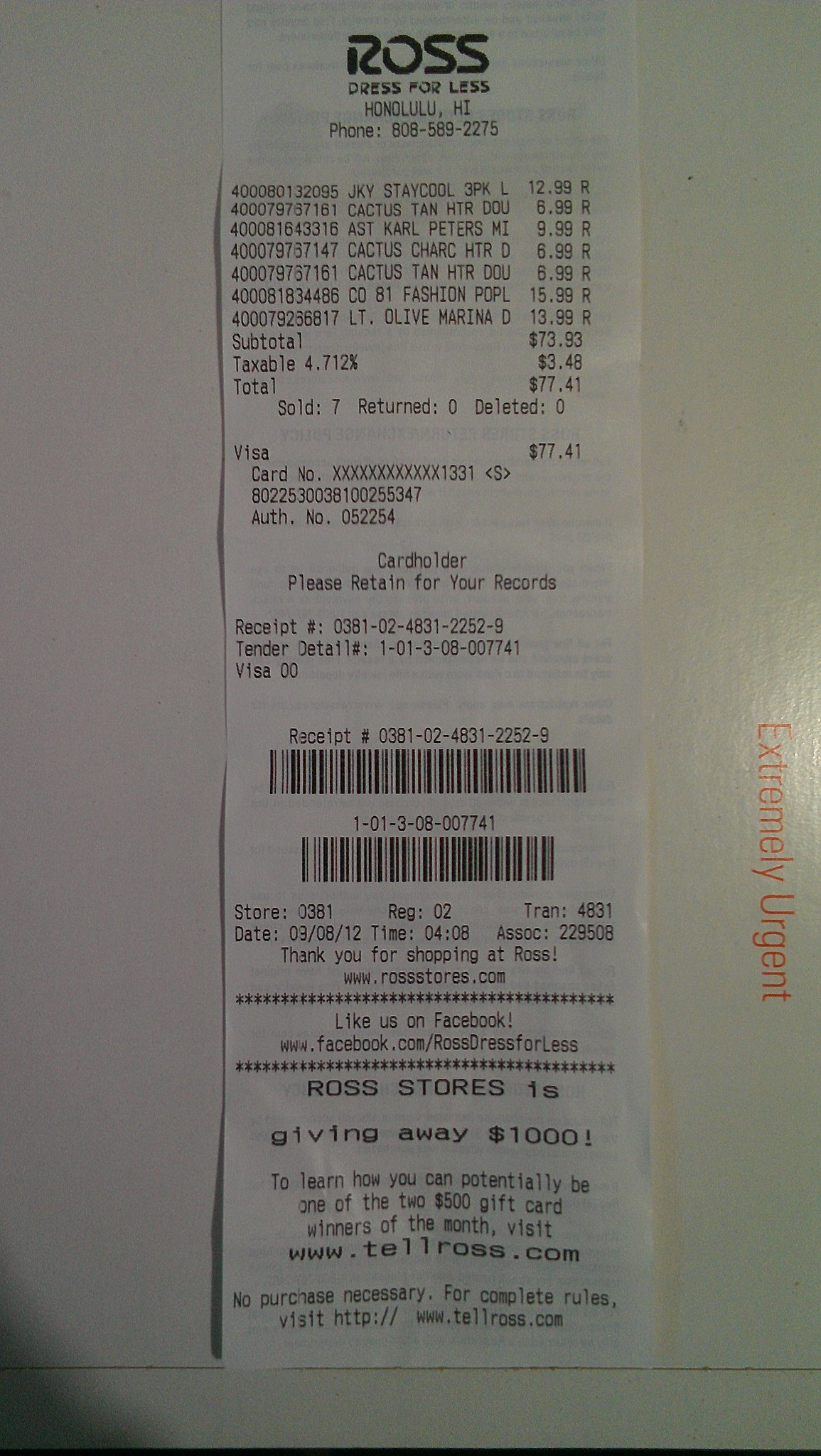A photograph displays a lengthy receipt strip attached to a white piece of cardboard with the phrase "EXTREMELY URGENT" prominently printed in red letters. This receipt is from Ross Dress for Less in Honolulu, Hawaii. The detailed breakdown to the right lists various articles of clothing along with their respective prices, culminating in a total amount of $77.41. The white cardboard shows light reflecting off the word "EXTREMELY," creating a shiny effect. In the bottom left corner, a shadow partially obscures the cardboard, adding depth to the scene.